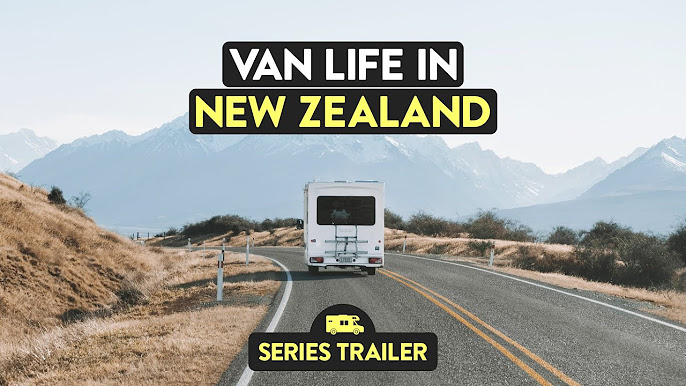This image, likely the cover of an advertisement or flyer, captures a picturesque outdoor scene in New Zealand. The top of the image features the text "Van Life New Zealand" in white and yellow against black banners, while the bottom reads "Series Trailer." In the foreground, a white van or RV is seen traveling along an asphalt highway marked with double yellow lines in the center and white lines on the edges. The road curves through dry, tan-colored grass to the left and stretches towards a distant mountain range under a clear blue sky. The sky is illuminated by the sun, casting a bright, inviting glow across the landscape. The overall scene is serene, highlighting a combination of open road adventure and natural beauty.